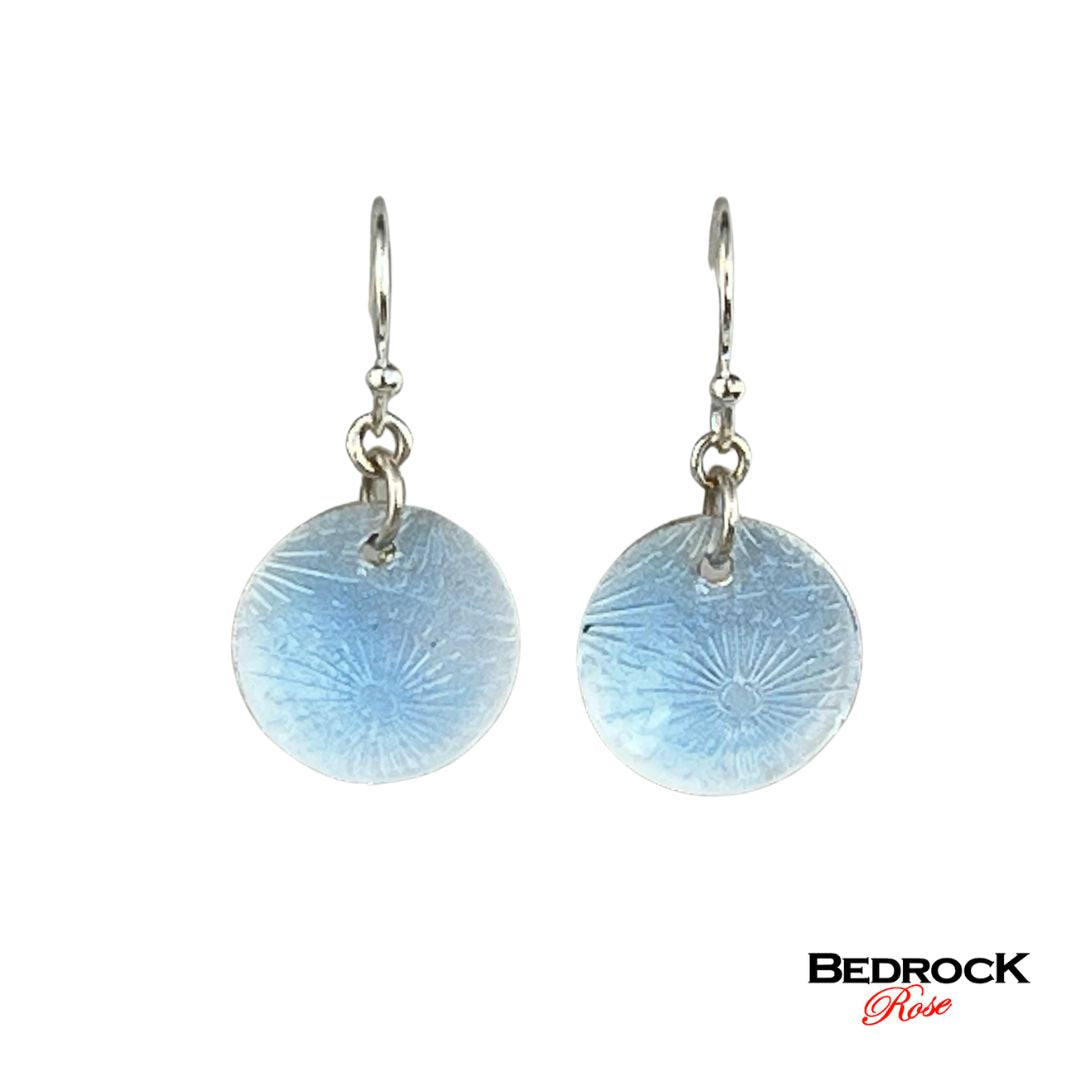This image is a detailed color photograph of a pair of silver, dangly earrings, set against a white background. Each earring features a silver hook at the top for securing in the ear. Below the hook is a small silver ball, followed by an interlocking series of silver circles and loops attaching to the main pendant. The pendants are circular and appear to be made out of a light blue, possibly glass or plastic material that has a shiny finish. The surface of the pendants is textured with faint designs that resemble a sun, featuring radiating lines or sun rays, and possibly include crater-like spots that give a celestial appearance, similar to the moon. At the bottom right corner of the image, the text "BEDROCK" is prominently displayed in black capital letters, and directly beneath it, in red cursive script, is the word "Rose," with a distinctive, ornate swirl on the capital "R".